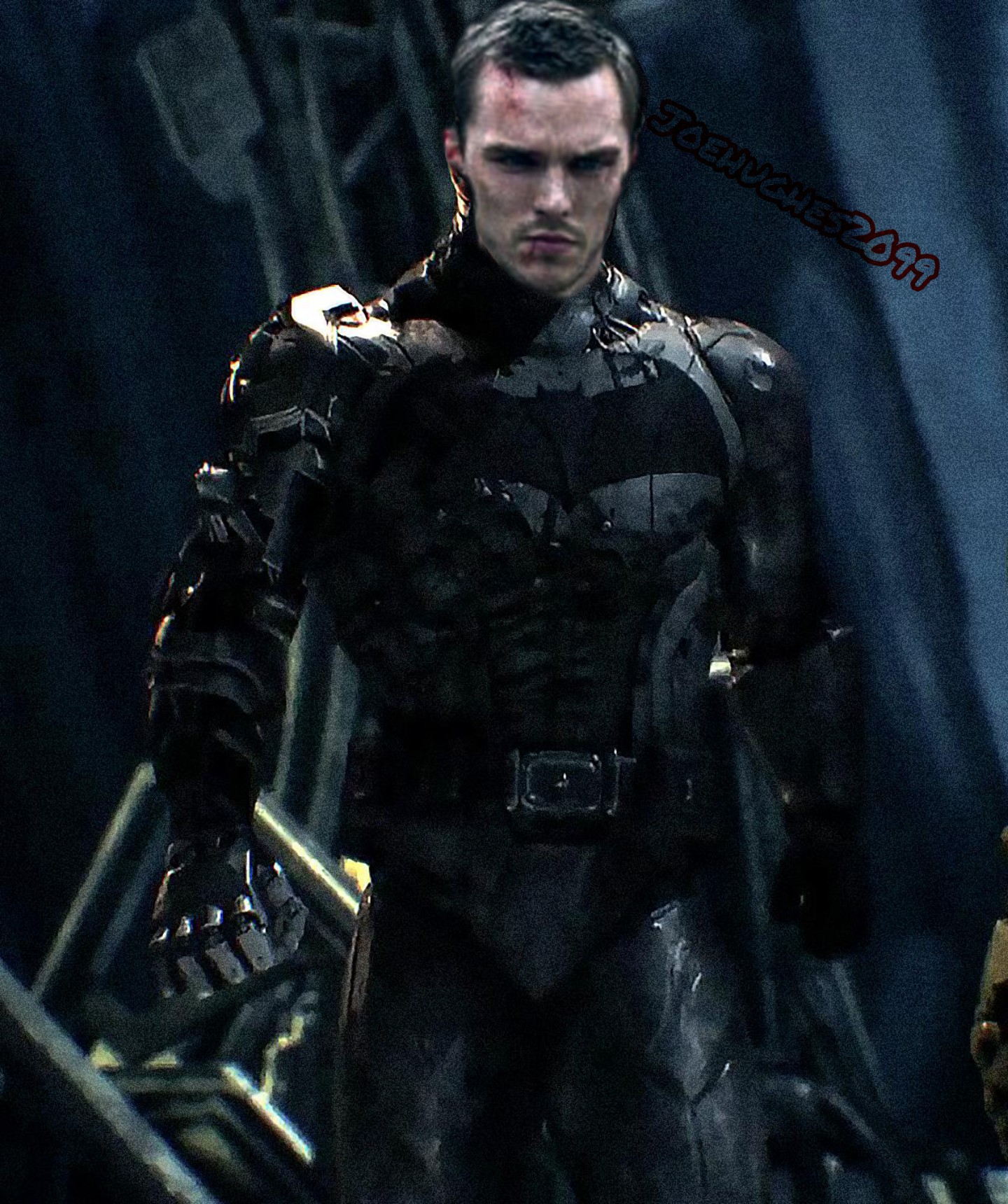In a dimly lit, dull-toned scene that seems to be set outdoors at night, the image features a man at its center, clad in an ultra-fit, black superhero outfit with silver and gray highlights. The suit, which appears plasticky, is meticulously designed with pronounced muscle cutouts that accentuate his biceps, triceps, shoulder muscles, and thighs, giving him a robust and powerful appearance. The outfit includes a belt at the waist and gloves that suggest strong, punch-ready fists, yet it leaves his face and hair exposed. The background appears to be the side of a building, shrouded in dark bluish tones. Across the top, angled diagonally from the middle to the right-hand side, is the text "Joe Hughes 2099," marking the image with a futuristic copyright.